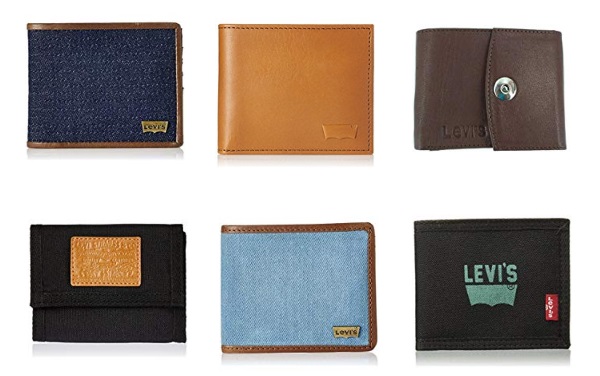The image showcases six Levi's brand wallets arranged in two neat rows on a plain white background, likely intended for display purposes. The top row features three wallets: on the left is a brown wallet with a navy blue border and the Levi's logo positioned at the bottom right; in the center is a tan wallet; and on the right is a brown wallet with a button in the middle, sporting the Levi's logo indented on the left. The bottom row also contains three wallets: the leftmost is black with an orange square that has text inside; the middle one has a light blue body with a brown border and the Levi's logo on the bottom right; and on the right is a dark gray wallet with Levi's written across the middle, accompanied by a small red Levi's tag. The wallets are presented in a simplistic yet organized manner, potentially for a store display or an online catalog.